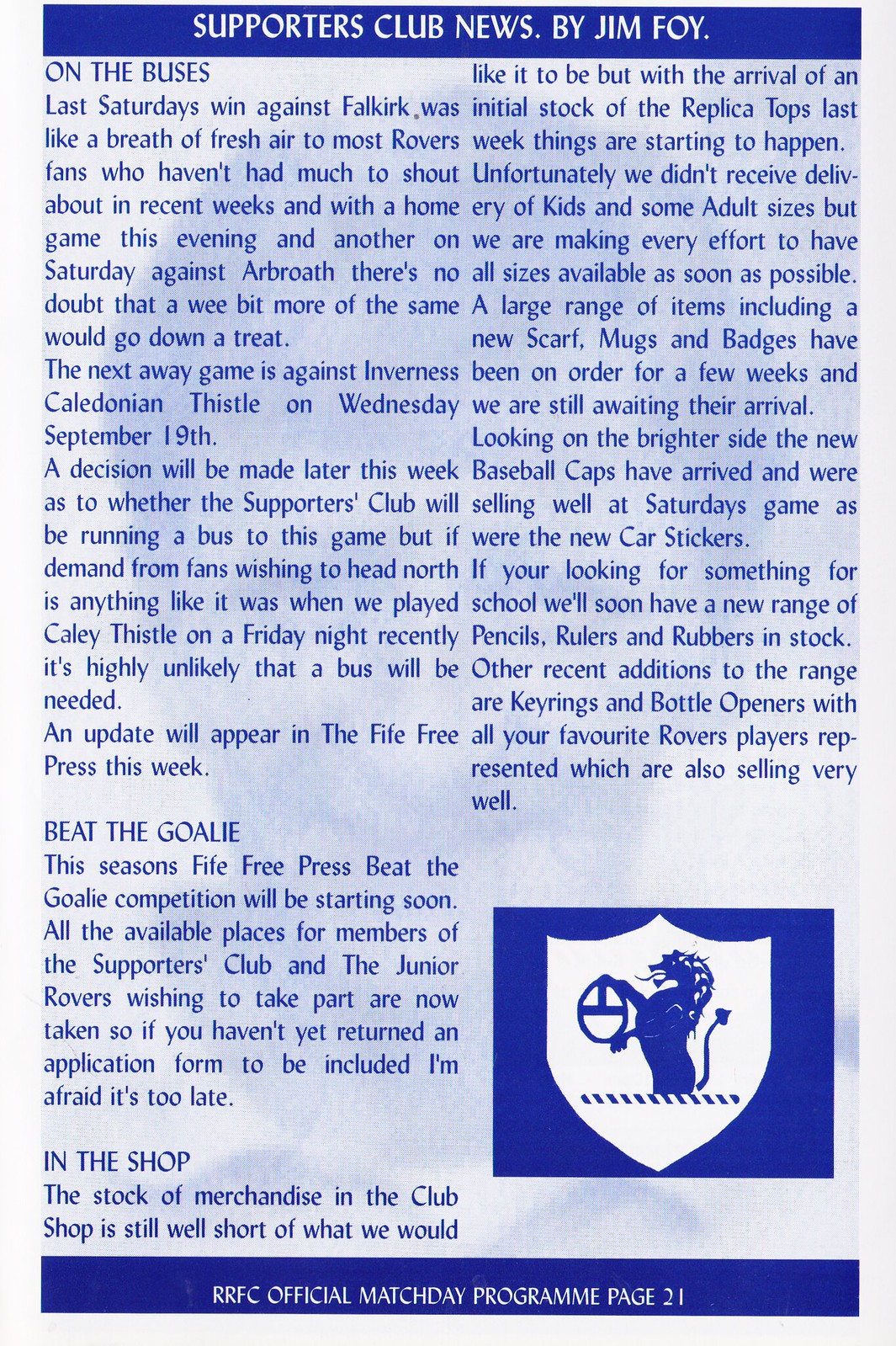The image is a tall, rectangular flyer with a light gray background featuring a light bluish-gray pattern. At the top, in white fonts over a dark blue rectangle, it reads "Supporters Club News by Jim Foy." The bottom of the flyer displays "RRFC Official Match Day Program, page 21" in white fonts over a similar blue rectangle. In the bottom right corner, there is a blue and white insignia overlapping a horizontal blue rectangle. The flyer is from a British football club magazine and has two columns of text. The first story is titled "On the Bus," discussing recent matches and future travel plans for the supporter’s bus. The second story, "Beat the Goalie," mentions an upcoming competition where all available spots are filled. The final section is called "In the Shop." The entire page has a blue hue with blue stripes and various blue-themed elements.